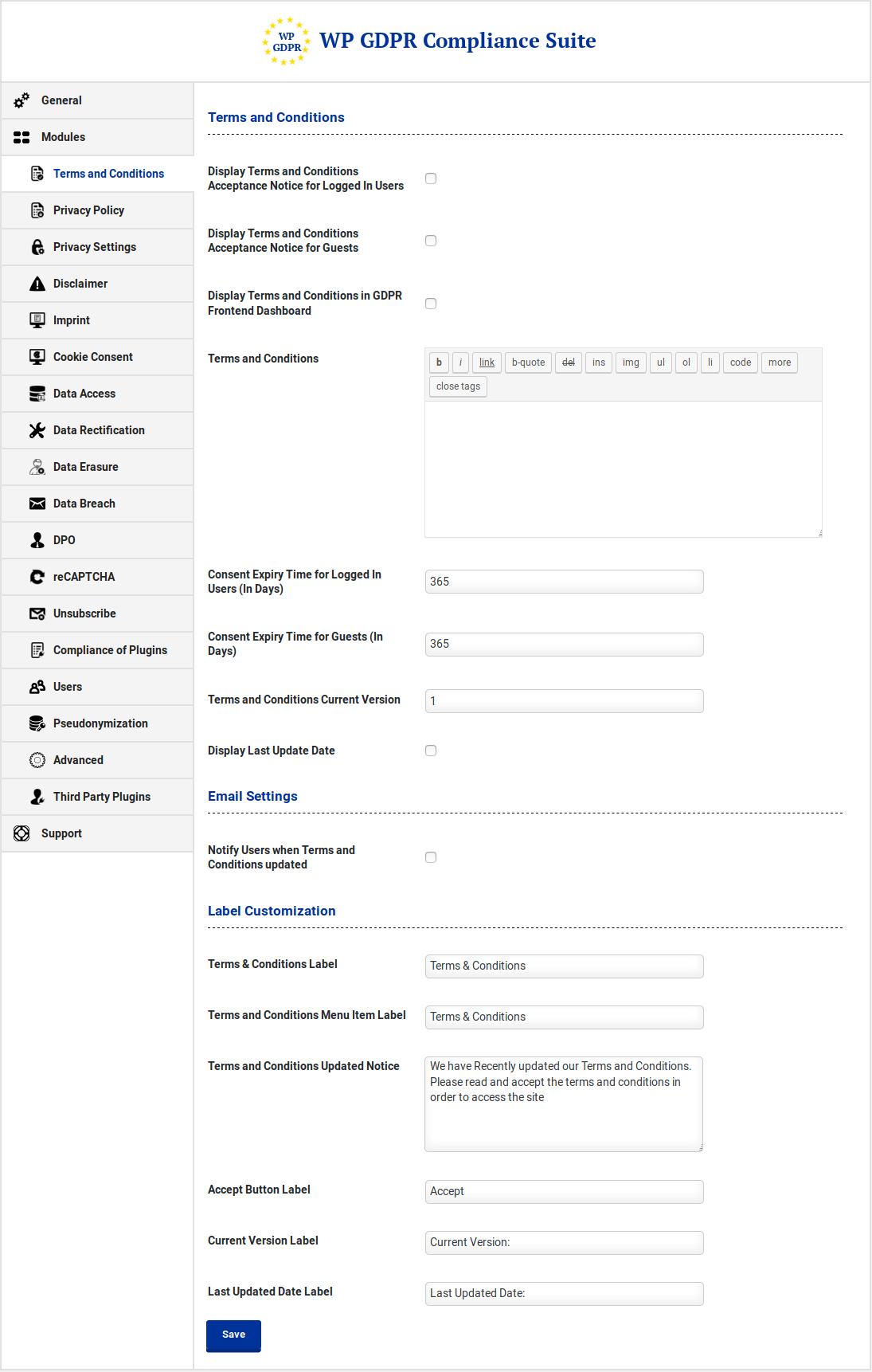Screenshot of a mostly white webpage featuring a gray column on the left-hand side. The column is titled "WPGDPR Compliance Suite" with "WPGDPR" in all caps and "Compliance Suite" in blue, lowercase letters. Below the title, the following text is listed in very fine print: 

- "Terms and Conditions"
- "Display Terms and Conditions Acceptance Notice for Logged in Users"
- "Display Terms and Conditions Acceptance Notice for Guests"
- "Consent Entry Time for Logged in Users (in days)"
- "Consent Expiry Time for Guests (in days)"

The tiny font makes the text difficult to read.